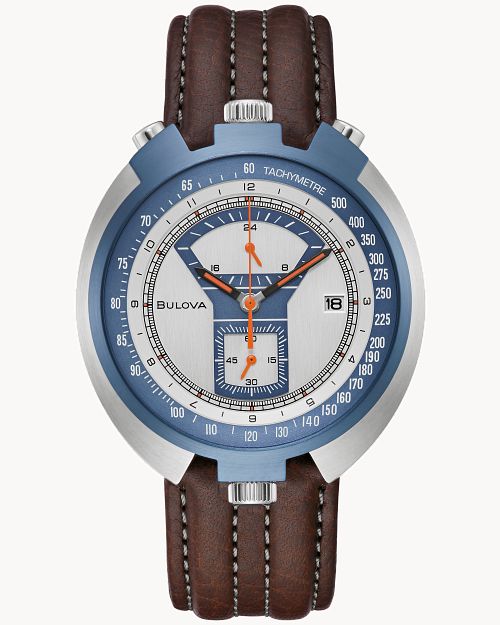The image showcases a detailed, high-end Belova watch. The watch features a dark brown leather band accented with light brown stitching. Its face is metallic with a combination of silver and medium blue tones. The outer edge of the watch face is blue with a series of numbers, indicating that it functions as a tachymeter, making it suitable for precise time and speed measurements. The inner watch face is silver, equipped with typical analog clock hands in black, and includes a date display. The second hand is distinct with a red-orange color. The watch also has three buttons on the top and one on the bottom, all in silver and likely adenized aluminum, which allows the user to set and adjust various features. The background of the image is pure white, emphasizing the professional, advertisement-like quality of the photograph. The watch is positioned head-on, displaying perfect clarity of its elegant and multifunctional design.